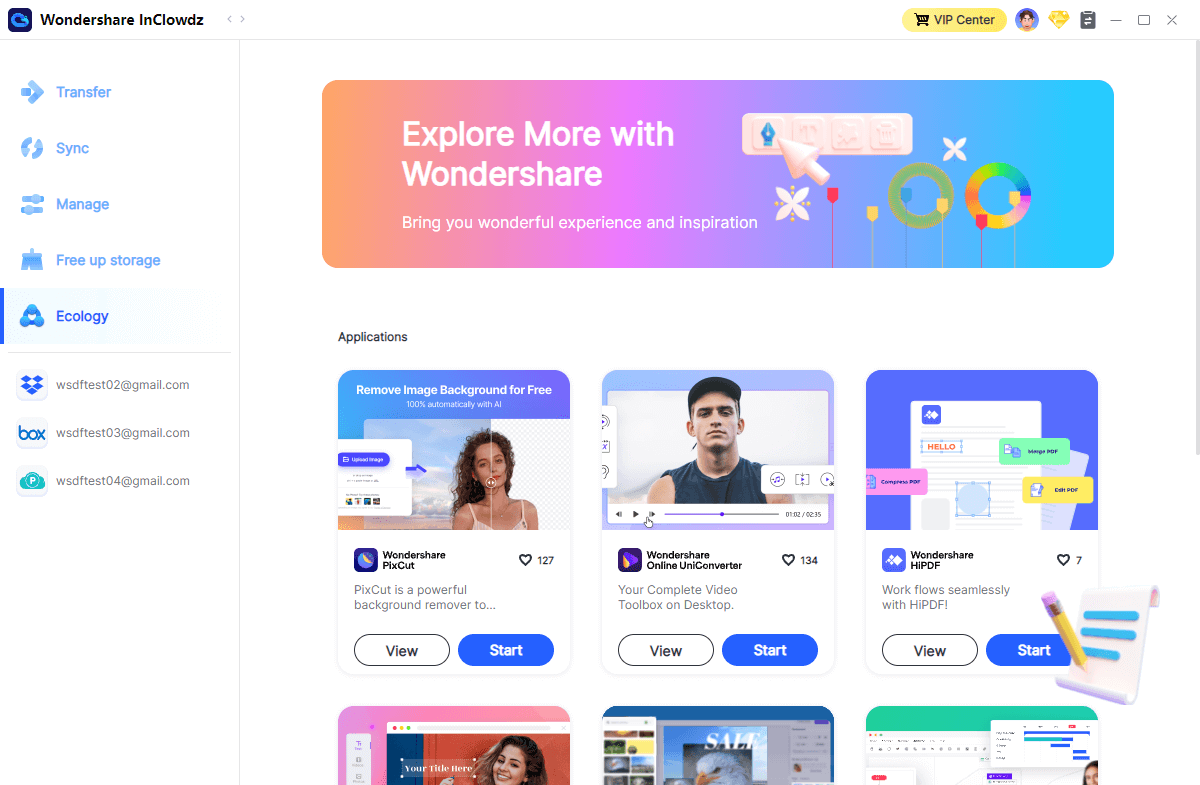The image depicts a webpage from a website called "Wondershare in Clouds," spelled with a 'Z' at the end. The layout features a light blue vertical menu on the left with options such as Transfer, Sync, Manage, Free Up Storage, and Ecology. The icons beside these options are also light blue, but the Ecology option is highlighted with a darker shade of blue, and a vertical blue bar to its left signifies it is selected. Below this menu, there are icons for cloud storage solutions like Dropbox, Box, and another marked with a 'P' inside a cloud, likely indicating additional storage services. 

Displayed on the main section on the right is a header adorned with arrows, circles, and floral graphics. The background of this section transitions from orange on the left to pink, then purple, and finally light blue on the right. The header text reads, "Explore more with Wondershare," accompanied by the tagline, "Bring your wonderful experience to end inspiration." 

Above this header, the top right corner exhibits a VIP Center icon, a user profile picture, and additional icons for closing and minimizing the window. Below the header, the page shows an 'Applications' section with three visible tiles. The first tile is for "Wondershare Pics Cut," a background remover, featuring an image of a woman with a beach background. The second tile mentions an online converter service shown with a white screen and a person, likely indicating video format conversion capabilities. The third tile is labeled "Hi PDF," suggesting tools for creating PDFs, represented with corresponding graphics. More tiles appear to be partially visible at the bottom of the image. 

Additionally, the page includes web addresses, such as wsdftest234 and gmail.com, implying individual user profiles or accounts.